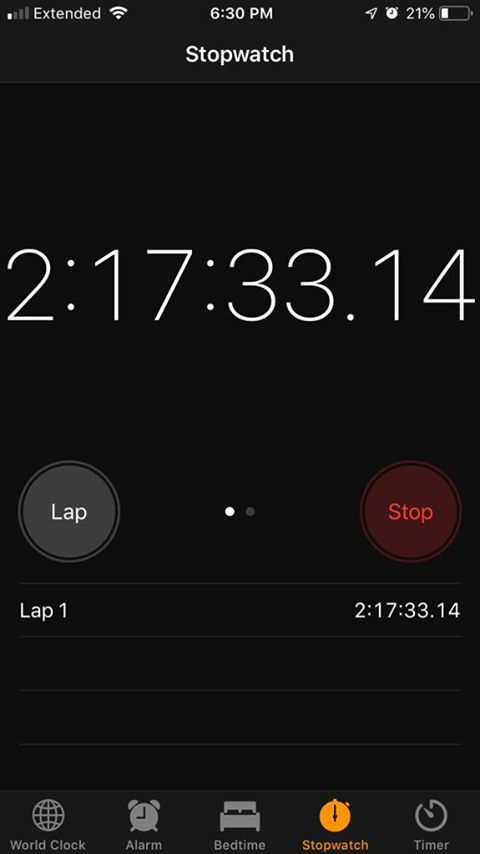A detailed screenshot of a stopwatch interface on a smartphone is depicted. In the upper left corner, the status bar contains icons indicating various statuses: network signal strength (or lack thereof), extended network availability, and full Wi-Fi strength. The time is displayed as 6:30 p.m., followed by icons for location services, an active alarm clock, and a battery indicator showing approximately 25% remaining charge.

The header for the stopwatch appears in white text within a black rectangle. Below this header, the time elapsed is prominently displayed as "2:17:33.14." Underneath the elapsed time, a grey circular button labeled "LAP" (in all capital letters) provides functionality for recording lap times. Two dots below the LAP button, with one white dot indicating the current page, offer navigation cues.

Towards the right side of the screen, a circular button with a blackish-reddish hue is labeled "STOP" in red text, ready to halt the stopwatch. Beneath this control area, a record shows "Lap 1" on the left, with the corresponding time of "2:17:33.14" on the right.

Further down the screen, a dark space leads to a row of additional buttons at the bottom. These include icons for a world clock, an alarm, a bedtime feature, a prominently highlighted orange stopwatch button, and a timer. Each of these options provides access to different time-related functions within the application.